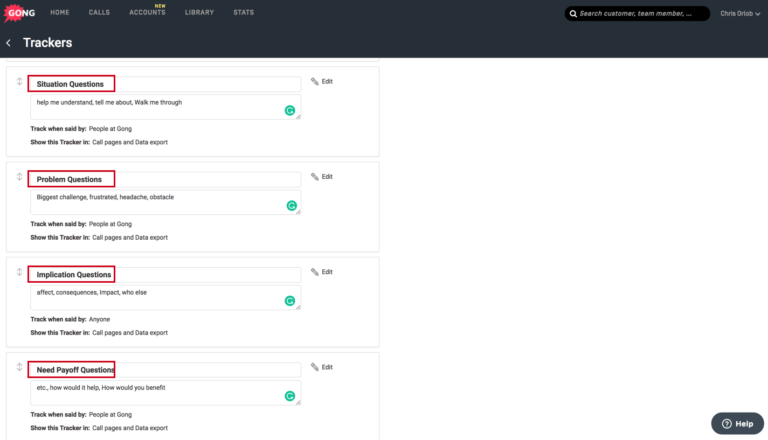In the image, we see an application or web page that is predominantly white in its design. At the top, there's a black navigation bar that stands out against the white background. In the upper left corner of this bar, the word "Gong" is clearly visible, accompanied by a red icon. The navigation menu includes buttons labeled Home, Calls, Accounts, Library, and Stats. 

To the right of the navigation menu, there's a search box with placeholder text. Additionally, there's a user section labeled "Chris Orlob," likely indicating the user's profile. Adjacent to this, the word "Trackers" is accompanied by a left-pointing arrow.

Below the black navigation bar, most of the page is white and features a series of questions divided into sections:

1. **Situation Questions**: This section includes prompts such as "Help me understand," "Tell me about," and "Walk me through." There’s a green Grammarly (G) icon next to text stating, "Track 1 said by people at Gong. Show the tracker and call pages and data export."

2. **Problem Questions**: Possible prompts here include "Biggest challenge," "Frustrated," "Headache," and "Obstacle," with corresponding text boxes for input below each prompt. 

3. **Implication Questions**: This section includes prompts like "Affect," "Consequences," "Impact," and "Who else."

4. **Need-Payoff Questions**: Prompts in this section read "How would it help?" and "How would you benefit?"

Each question category has an associated chat box where responses can be typed in. At the bottom right of the page, there is a black button labeled "Help."

The overall layout is clean and structured, with each section clearly demarcated, allowing for ease of navigation and interaction.